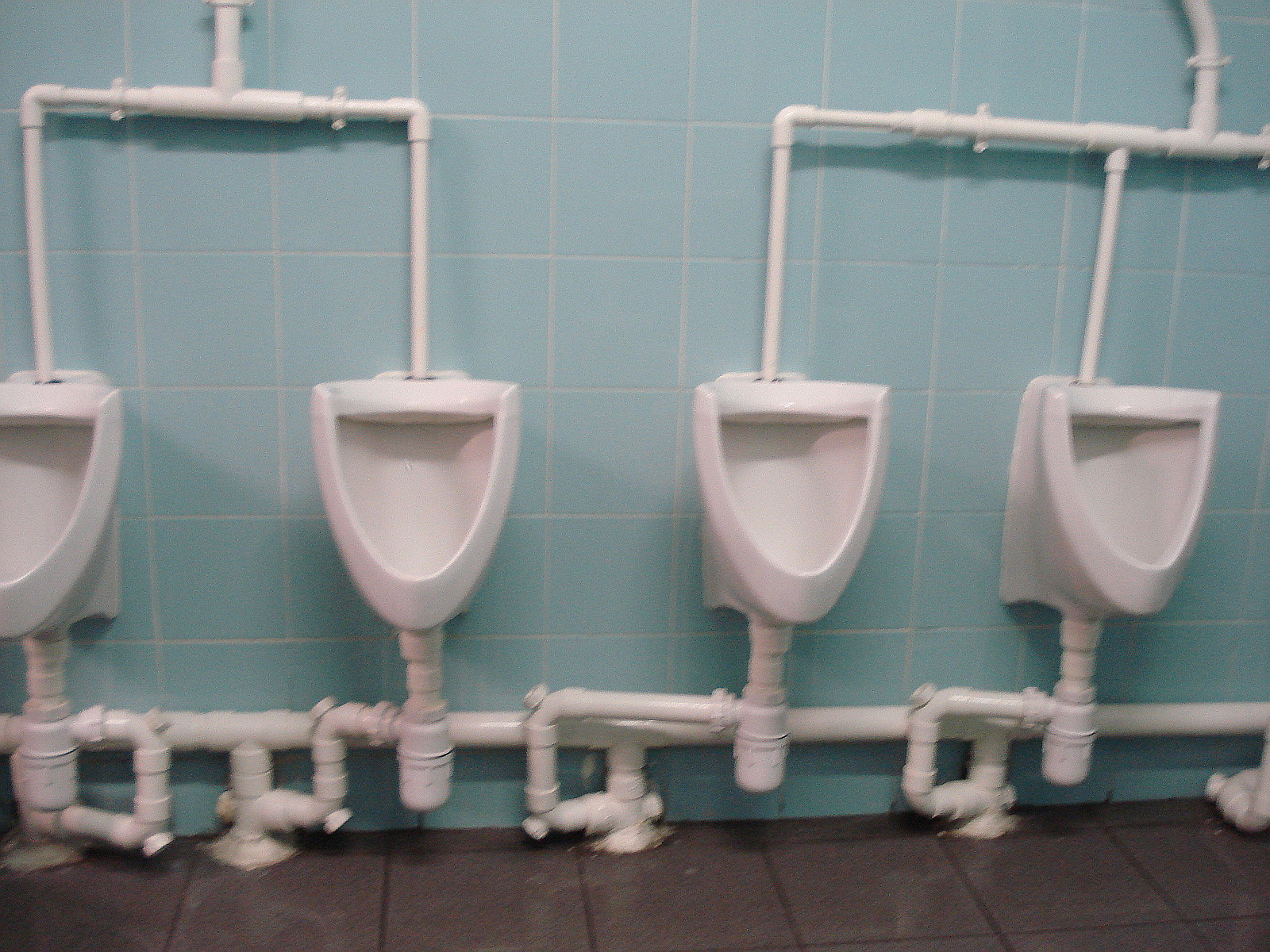This is an indoor color photograph showcasing a row of four white ceramic urinals mounted on a wall covered with large, square blue tiles. The urinals are evenly spaced and feature an elaborate array of exposed white PVC piping both above and below them. The upper pipes feed water into the units, branching off to service pairs of urinals. The bottom pipes manage the drainage, forming an intricate network of vertical and horizontal lines as they connect to a longer pipe near the dark brown tiled floor. The piping is visually prominent as it is not concealed within the wall, giving a stark, industrial feel to the otherwise modern and bare-bones design of the urinals. The units appear to be self-flushing, as there are no visible flush handles or automatic sensors present. The photograph is slightly grainy and somewhat out of focus, adding a raw, unpolished element to the scene.